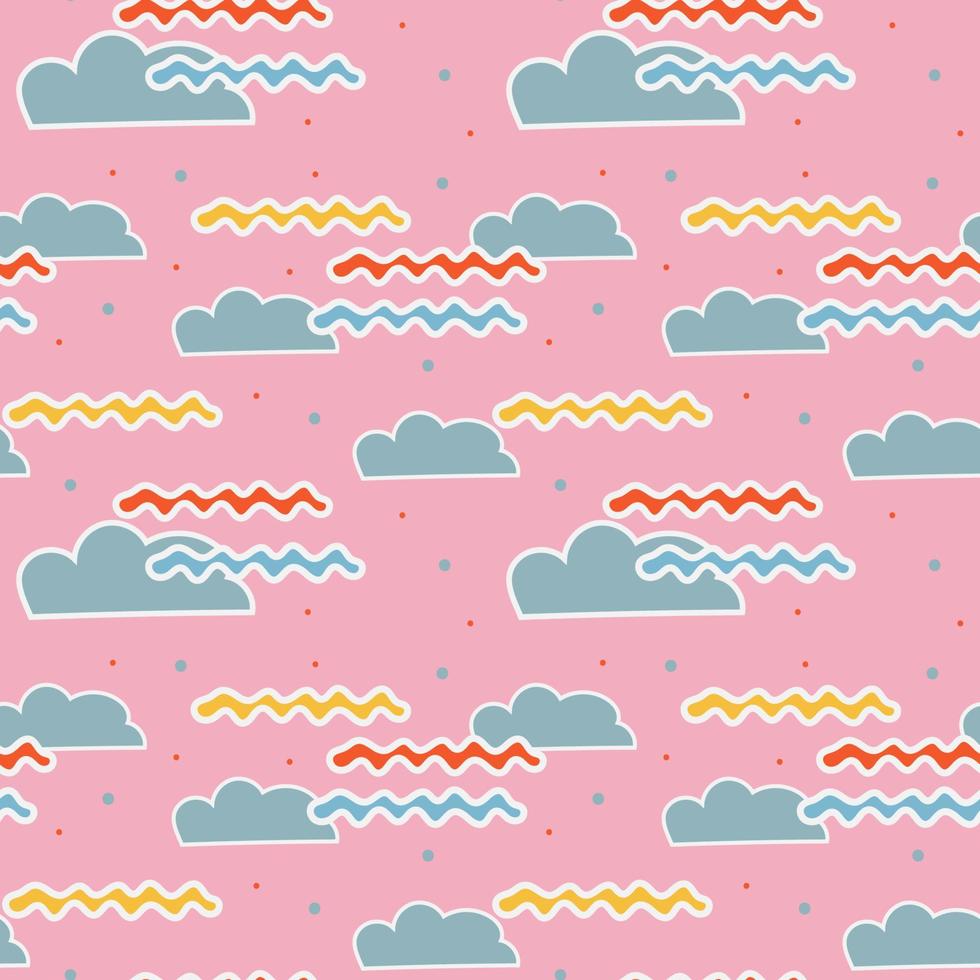The image features a square piece of light pink background, adorned with whimsical decorations that give it a vibrant, youthful quality, reminiscent of nursery designs. Scattered across this background are approximately 15 greenish-blue clouds, each outlined in white, varying slightly in size and seemingly angled as if drifting to the left. These clouds are interspersed with clusters of colorful squiggly lines—red, yellow, and the same greenish-blue as the clouds. The wavy lines resemble crudely drawn shoestring french fries and alternate between the colors, positioned above and below the clouds, with the greenish-blue ones extending from the clouds themselves. Additionally, the pink background is sprinkled with red and greenish-blue polka dots, with the blue dots larger than the red, adding a playful sprinkle effect. This dynamic design evokes a sense of motion and energy, making it perfect for a child’s nursery or playful wrapping paper.